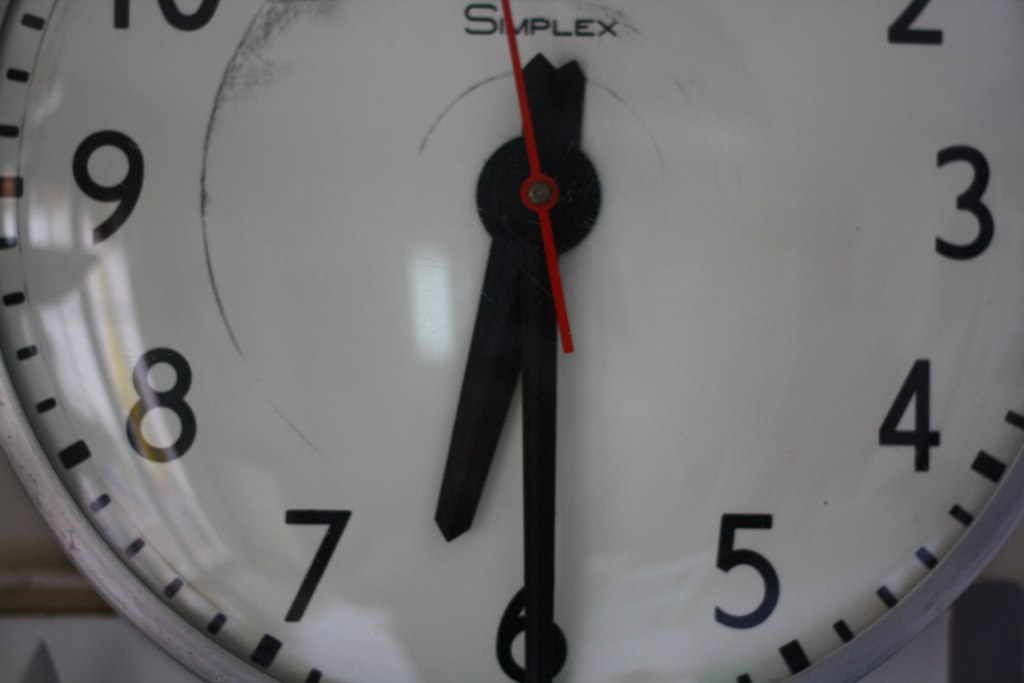This close-up photograph captures a partially visible face of a Simplex-branded wall clock with a worn white surface. The clock's time is set to 6:30, indicated by two black hands for the hour and minute, and a thin red hand for the seconds. The image highlights the numbers from 3 to 9, while only parts of 10 and 2 are visible. The clock's silver rim is evident in the bottom corners. The face shows signs of wear, with faint, scratched circles marking the paths of the hands. Black numbers and minute markers are prominently displayed, contributing to the clock's slightly aged appearance.